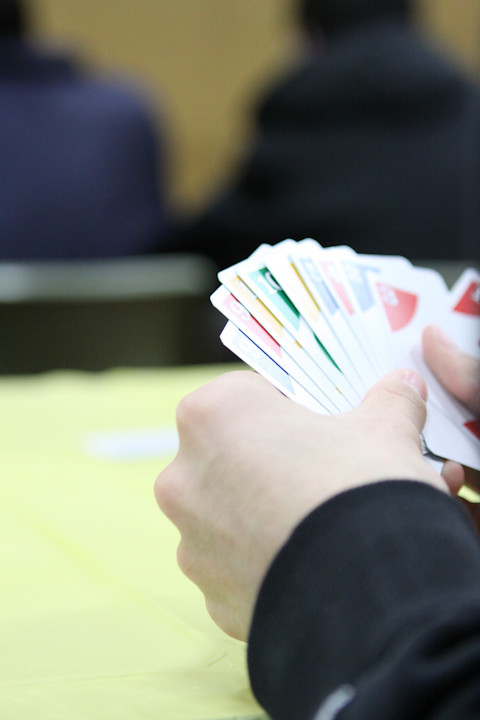In this photograph, a classroom setting is depicted, though the background is notably blurry. The main focus is on two individuals seated at desks, viewed from the back. The person on the right is wearing a black hoodie and has black hair, while the person on the left is donned in a blue jacket. In the foreground, the arms and hands of another individual are visible as they hold a hand of cards, which appears to be a deck of Uno cards. The subject's left hand is prominently shown up to the knuckles, with the thumb and part of the deck. The right hand's thumb and pinky finger are also visible, indicating a grip on the cards. This person is wearing a black jacket, and their arms are resting on a table covered with a yellow tablecloth. The scene suggests a casual and collaborative environment, possibly during a break or a recreational activity within the classroom.